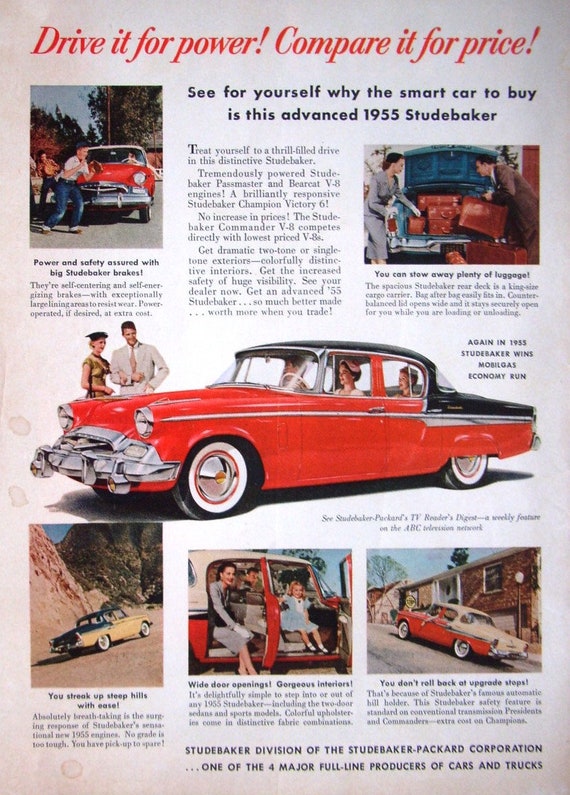This vintage advertisement, likely a magazine page from 1955, promotes the advanced Studebaker car. Dominating the top are bold red phrases, "Drive it for power! Compare it for price!" Beneath this, in black letters, it declares, "See for yourself why the smart car to buy is this advanced 1955 Studebaker." Various images of the car adorn the advertisement: a prominent red model with a black top and a touch of grey, and other versions including a red car with a beige back, and a beige car with a dark green or blue back. 

One central image showcases a woman driving with a man beside her and a child in the back seat. Surrounding this, additional scenes depict a variety of uses: a boy with a baseball glove in front of the car, a man and a woman packing the trunk with suitcases for a trip, and a woman and a girl with the car doors open. The bottom left shows the car effortlessly ascending a hill with the caption, "You streak up steep hills with ease," and another image confirms its stability parked on a hill.

The advertisement further emphasizes the car's accolades, noting the 1955 Studebaker's victory in the Mobilgas Economy Run, highlighting its power and safety features, and concluding with a nod to the Studebaker-Packard Corporation as a major car and truck manufacturer.